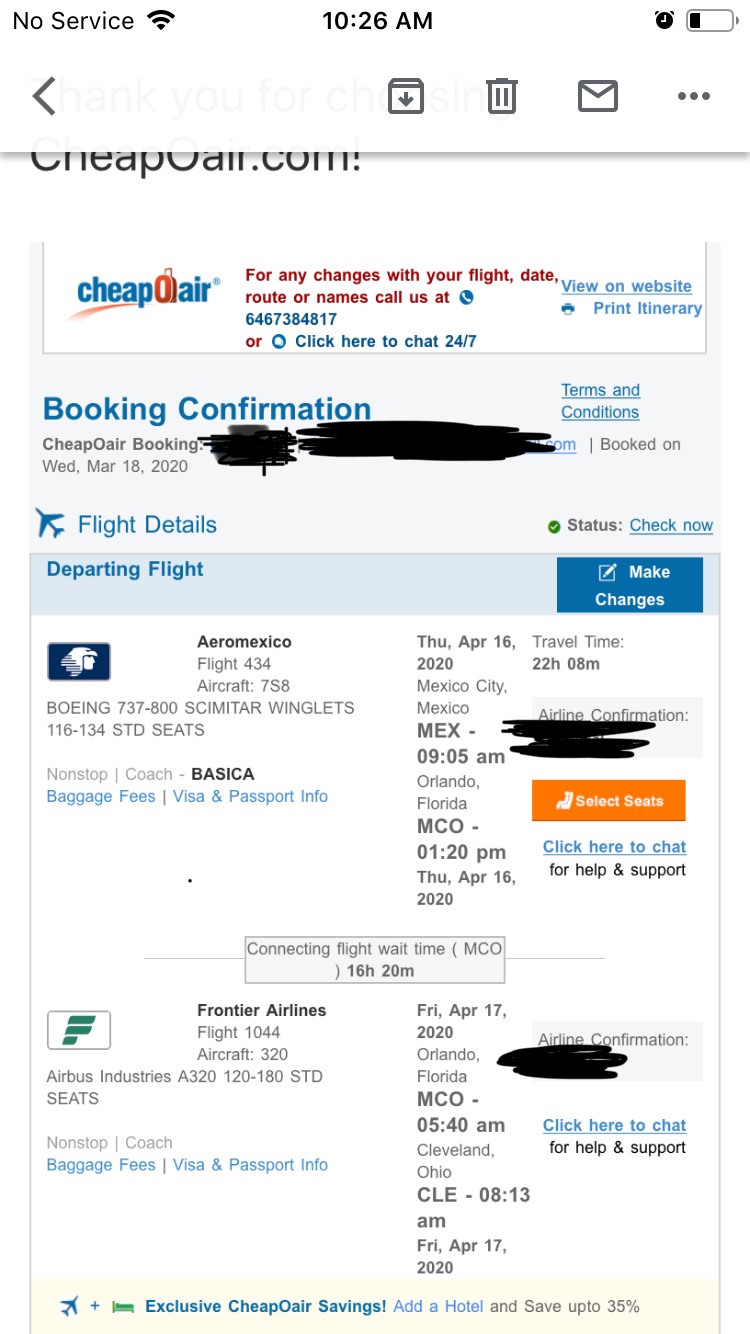A close-up photo of a cell phone screen displaying a flight itinerary from CheapoAir.com. The top of the screen shows the phone's status bar, indicating a low battery at around 20%, no cellular service, and the current time as 10:26 a.m. The image prominently features the CheapoAir.com logo twice. Beneath a message that reads, "For any changes to your flight data, route, or names, call us at [phone number] or click here to chat 24-7," are options to "View on Website" and "Print Itinerary." The booking confirmation area is scribbled out, likely with a black marker, for privacy reasons. The screen further includes a section labeled "Flight Details," listing the departing flight with Aeromexico on a Boeing 737 with split scimitar winglets. Seat information is provided, mentioning the class "BASICA." The bottom of the screen notes a Frontier Airlines flight 1044, along with additional flight-related information.